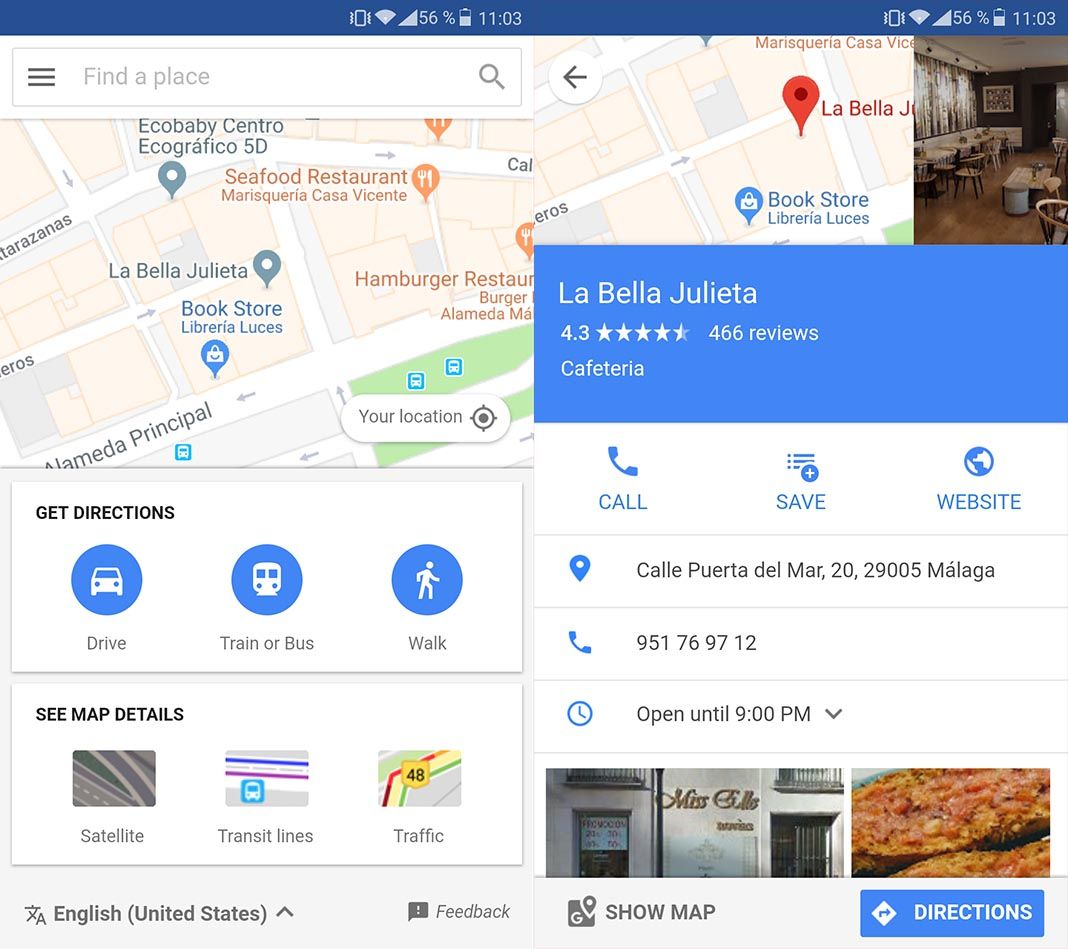The image depicts the user interface of a map application. In the top left corner, there is a search bar that prompts the user to "Find a place." Below the search bar, a detailed map is displayed featuring various establishments, including a seafood restaurant, a hamburger restaurant, a bookstore, and an establishment named La Bella Giulietta. 

On the right side of the screen, there is a blue rectangle highlighting La Bella Giulietta which is noted to be a cafeteria. It has a rating of 4.3 stars from 466 reviews. Adjacent to this information, in the top right, there is a photograph showcasing the dining room and the restaurant's exterior.

In the bottom left section of the interface, there is a button labeled "Get directions." Below this, three blue circles offer different modes of transportation: driving, taking a train or bus, and walking. A link titled "See map details" is present, which provides additional options such as viewing a satellite image, transit lines, and current traffic conditions.

To the right of the "Get directions" button, there are three icons labeled "Call," "Save," and "Website." Further details include the restaurant's address at Cali Puerto del March 20, 29005, a phone number, and its operational hours indicating that it is open until 9 PM. Below this contact information, two additional pictures are displayed.